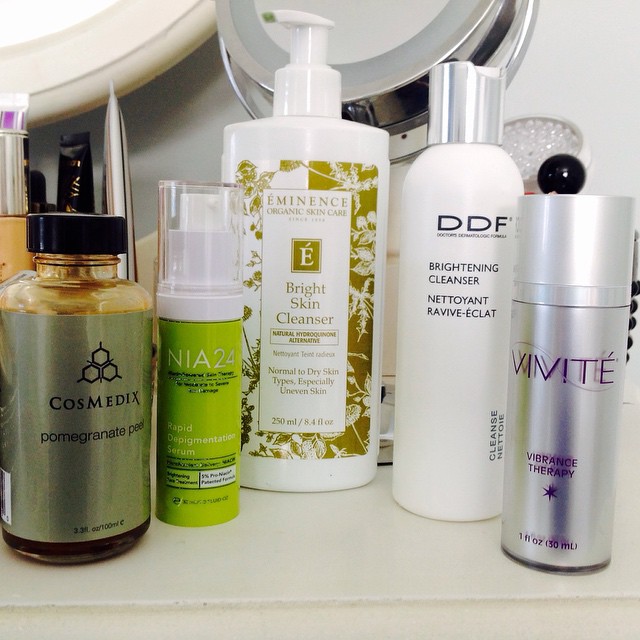This close-up image captures a neatly arranged bathroom countertop set against a white backdrop. The countertop is pristine white, which contrasts with the silver and white frame of a face mirror and wall mirror in the background, only partially visible. A series of skincare products dominate the foreground, moving from left to right. 

On the far left stands a bottle labeled "Cosmetics Pomegranate Peel." Next to it, a green container with a pump top reads "NIA 24 Rapid Depigmentation Serum," hinting at its role in skincare routines. The third item is a white bottle of skin cleanser, essential for daily cleansing. Neighboring this is another cleanser from the brand DDF, specifically a brightening cleanser. Finally, a product from VIVITE, likely a facial moisturizer, completes the assortment. Each item is meticulously placed, reflecting a well-organized and carefully curated skincare regimen.